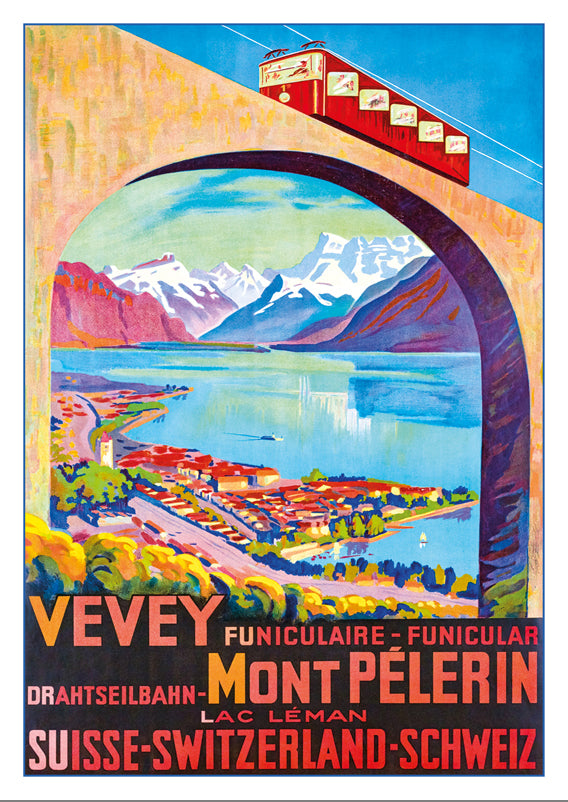The image is a vibrant and artistic poster with a cartoonish style, featuring a bustling, scenic landscape. Central to the composition is an enormous bridge with a substantial archway, made of brown, light-brown cement. Atop the bridge runs a red cart, resembling a small train, gliding along wires with people visible through its windows. In the background, beyond the bridge's arch, majestic snow-capped and regular mountains rise against a vivid blue sky tinged with yellow clouds. Below, a clear, blue lake reflects the grandeur of the landscape, bordered by a picturesque town with brightly colored buildings and lush trees. The text on the poster reads “Vivez Funiculaire, Funiculare, Dratsalbon, Mont Pelerin, Lac Le Mans, Suisse, Switzerland, Schweiss,” emphasizing its Swiss heritage. The overall palette boasts an array of bright blues, pinks, reds, and purples, making the scene both lively and eye-catching.